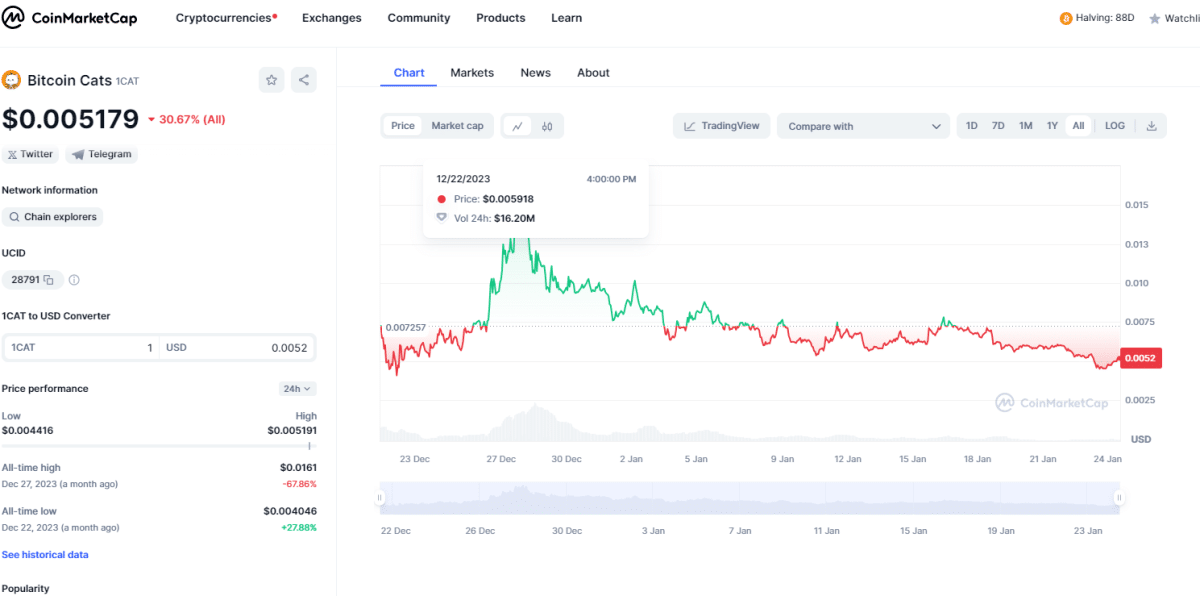**Screenshot from CoinMarketCap: Detailed Breakdown**

The image depicts a screenshot from CoinMarketCap, a popular cryptocurrency tracking platform. The interface features a prominent 'M' logo encircled, emblematic of the CoinMarketCap brand, stationed to the far left.

To the right, tabs are segmented for user convenience:
- **Cryptocurrencies:** Marked with a red asterisk.
- **Exchanges:** Proffers trade platforms.
- **Community, Products, Learn:** Sequentially positioned, guiding users through various sections of the site.

In the top-right corner of the interface:
- **Watchlist:** Represented by a star icon.
- **Halving (HU):** Displayed as "HALVING: 880" with a distinct orange icon adjacent to it.

Beneath the main CoinMarketCap header on the left:
- **Search Bar:** Here, 'Bitcoin Cash' is typed in, indicated as "Bitcoin cats one cat."
  - Next to it, star and share icons permit saving and sharing.
  - The current price flies at $0.005179, highlighted in red with a decline of -30.67%.

Further down, additional metrics and tools are available:
- **Twitter, Telegram Network Information**
- **Chain Explorers:** Allowing blockchain navigation.
- **ID:** Displayed with a corresponding number, though unclear in purpose.

A detailed section showcases:
- **Price Performance:** Offering toggles for performance views over 24 hours or other specified durations.
  - Featuring stats on high and low values and all-time highs.

To the right, the interface includes:
- **Chart, Market News, About Section:** Currently displaying a detailed chart.
  - The chart delineates market movement with red and green lines:
    - **Red:** Indicating performance operating at or below zero.
    - **Green:** Reflecting higher, positive performance.

The chart provides a temporal analysis from December 23rd through January 24th, offering extensive insights into the cryptocurrency's market behavior.